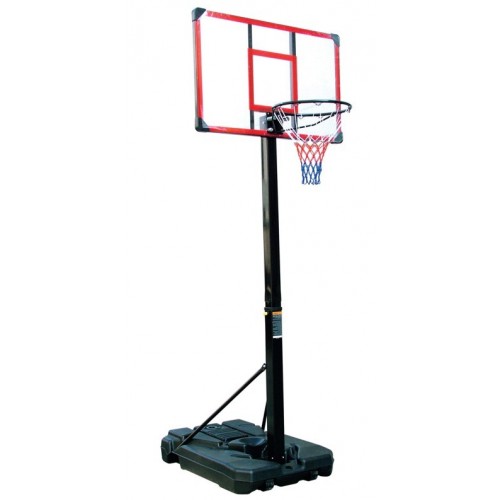The image depicts a modern basketball hoop positioned in the center against a pristine white background, reminiscent of a product advertisement one might encounter on retail sites like Walmart or Amazon. The hoop is presented at a slight diagonal angle, providing a partial side view. The setup features a durable black plastic base designed to be filled with water or sand for stability, and it includes wheels for easy mobility. Bracing supports extend from the base to the main pole, ensuring additional sturdiness. The pole itself is accompanied by a small, unreadable sticker. 

At the top of the pole, a transparent backboard is outlined with red and black markings, including a prominent red square in the center and two black lines. The backboard's corners are black while the rest of it appears clear, enhancing its modern look. The hoop features a black rim and a net with a striking red, white, and blue tricolor pattern. The equipment appears brand new and is in excellent condition, reflecting a high-quality product suitable for home basketball setups.